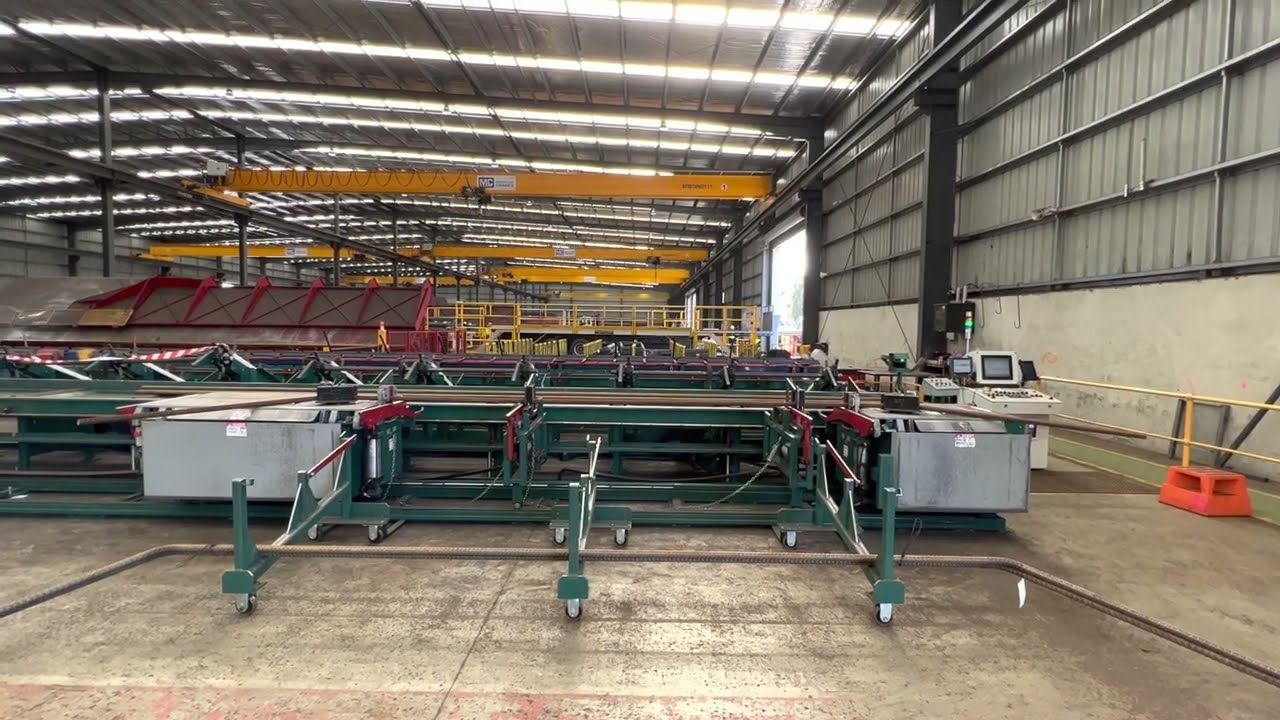The image depicts a vast, industrial warehouse or manufacturing facility characterized by extensive metal structures and equipment. The large, open space is dominated by long rows of green metal platforms or tables, intersected with wires and various machinery. Towards the right side of the image, there is a prominent black-framed computer with an adjoining cream-colored smaller screen and a keypad situated on a white podium with black keys. The ceiling is composed of metal roofing, supported by horizontal bars and beams, accompanied by pipes and interspersed with lighting fixtures. Yellow structural components and platforms hang from the ceiling, while a red stepstool is visible at the bottom right. In the background, large garage doors open to the outdoors, indicating it's daytime. The rear of the warehouse extends far back, featuring similar industrial equipment and a semi-truck trailer parked inside, further highlighting the expanse and operational nature of this facility.